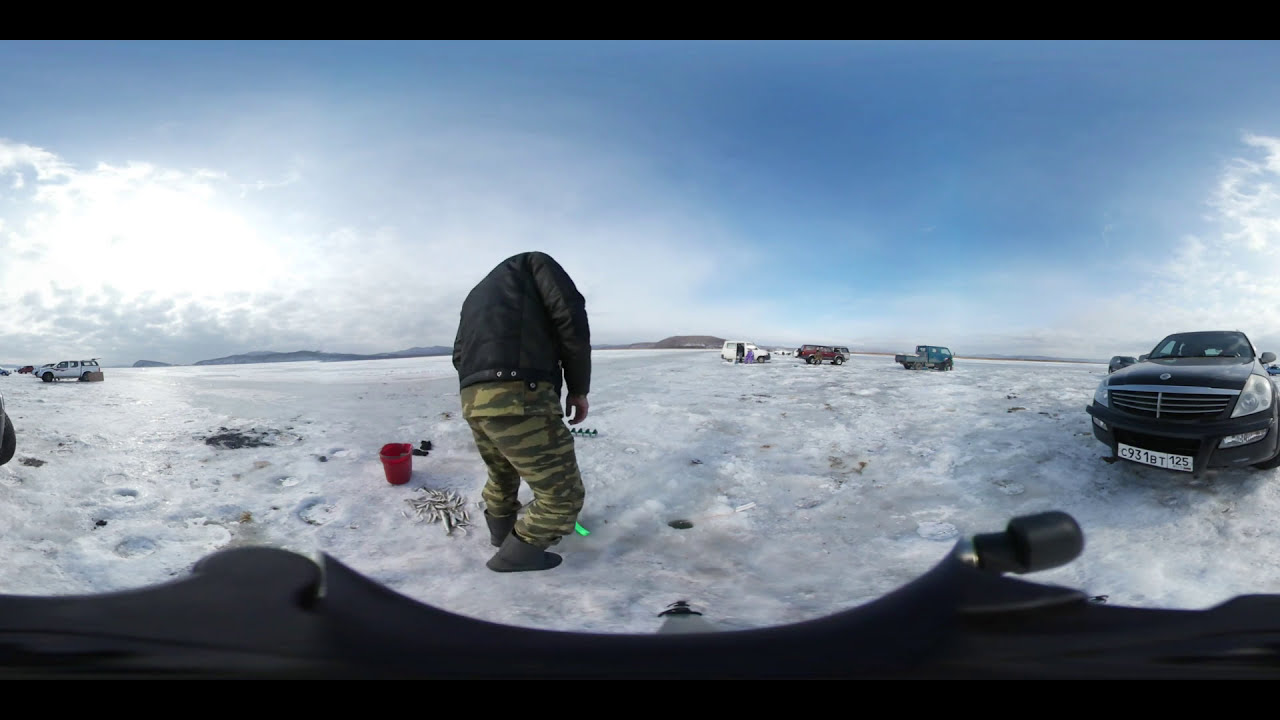In this detailed photograph taken outdoors in a cold, snowy environment, a man is preparing to go ice fishing on a frozen lake. The scene is marked by a blue, mostly clear sky with some clouds encroaching from the left. A black sedan, possibly with an Eastern Bloc or Russian license plate, is parked on the snow near the gentleman, whose attire consists of a dark black jacket, green camouflage pants, and dark boots. He stands near a small, freshly drilled hole in the ice, created with a gas-powered drill that rests on the ground beside him. Nearby, there is a red bucket and a small pile, likely of fish. In the background, three trucks and an additional car can be seen in the distance. The photograph seems to have a slight warping effect, indicating it may have been captured with a 360-degree camera, and some camera equipment appears to be slightly visible at the bottom of the frame.